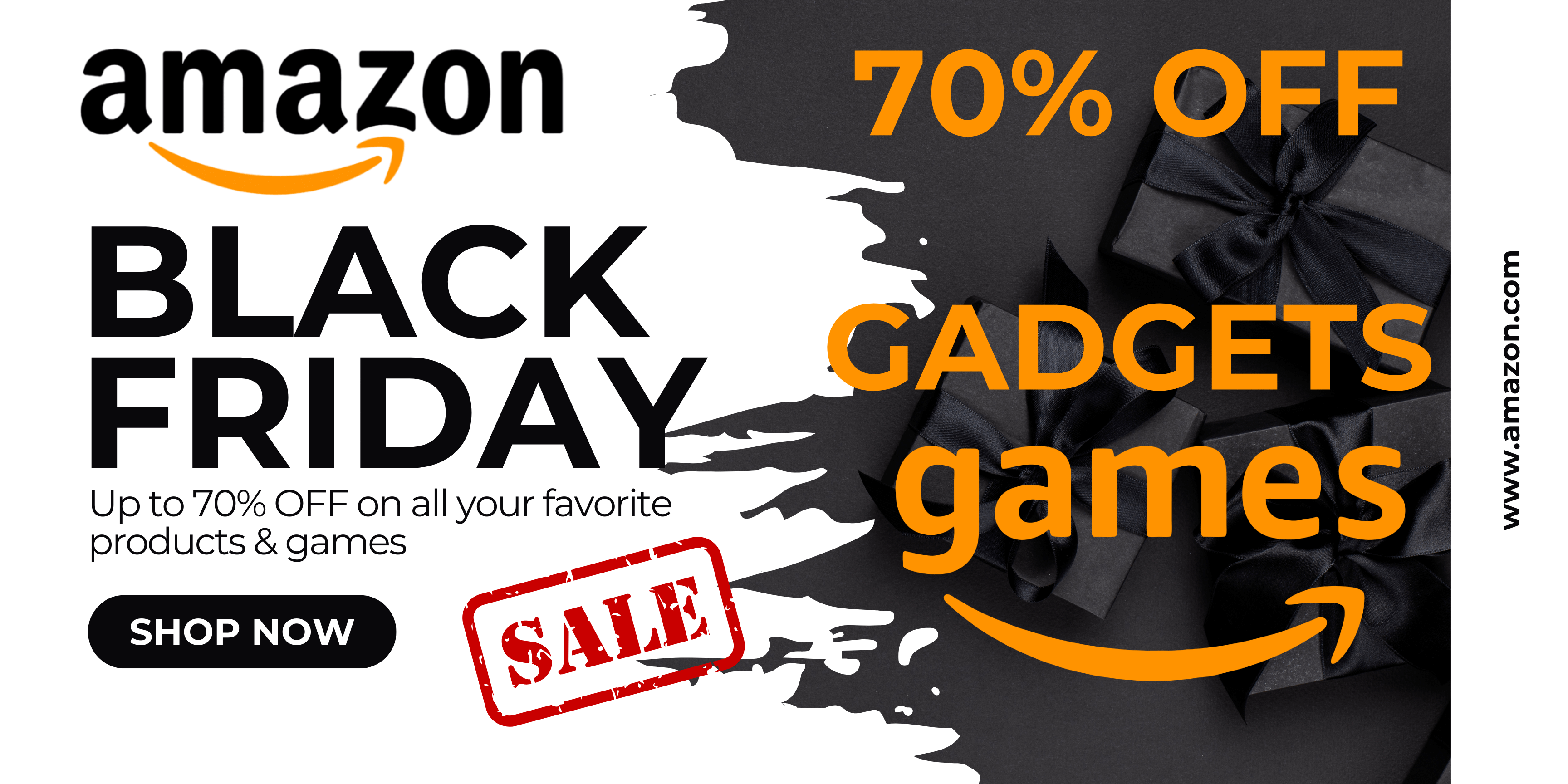This web advertisement for Amazon promotes their Black Friday sales event. Dominating the left side of the ad is the Amazon logo with the iconic curved arrow, accompanied by bold text that declares "Black Friday." Beneath "Black Friday," smaller text informs viewers that they can enjoy discounts of up to 70% on their favorite products and games. A prominent black button with white text reading "Shop Now" invites users to start shopping immediately through the provided link.

The right side of the advertisement contrasts with a black background featuring a watermark-like pattern of gift boxes. Overlaying this backdrop, bold orange text announces "70% off" in a striking splash font, with additional orange text beneath listing "gadgets" and "games" as part of the sale. Below, the Amazon logo with its signature curved arrow is displayed in orange. Finally, the far-right side of the ad includes the Amazon website, www.amazon.com, in black font against a white background, directing viewers to the shopping site.